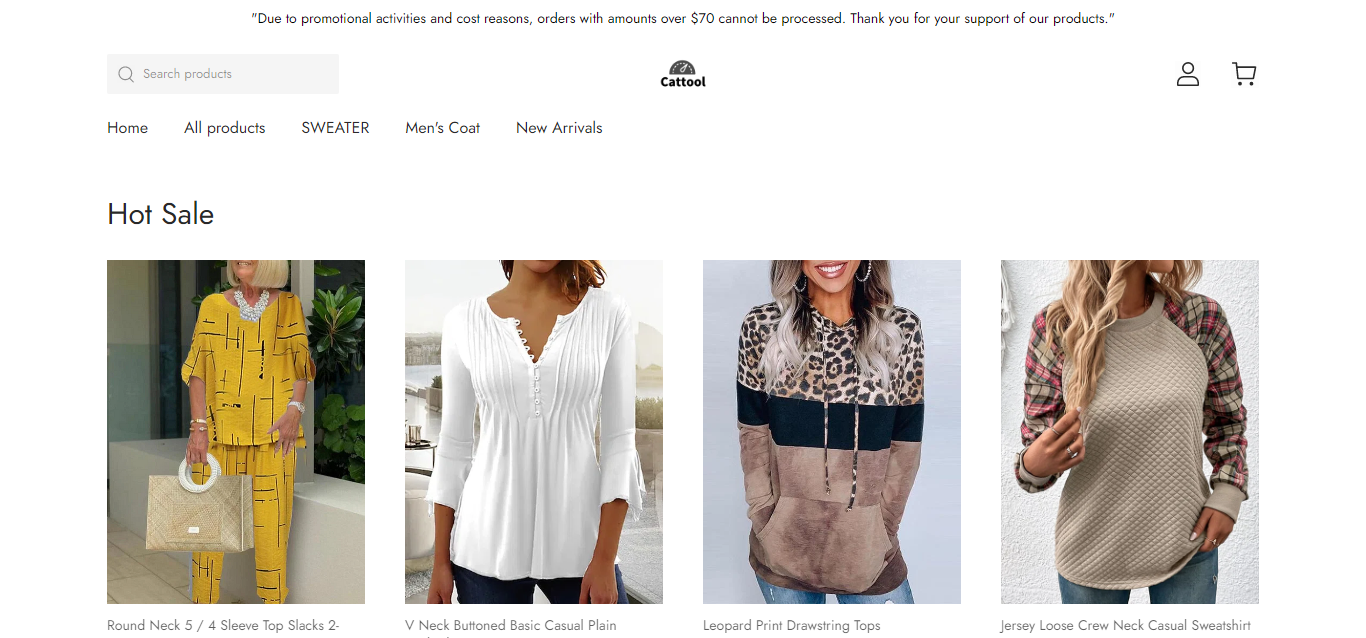The top section of the image features a stark white background with a black strip along the top, adorned with a quotation reading, "Due to promotional activities and cost reasons, orders with amounts over $70 cannot be processed. Thank you for your support of our products." On the right side, outlined in black, are icons of a person and a shopping cart.

Centrally positioned, the text "CAT2" is displayed above a gray progress meter. To the left of this, a gray rectangle houses a gray magnifying glass icon accompanied by the words "Search products." Below this search bar are navigation links in black reading: "Home," "All Products," "SWEATERS," "Men's Coats," "New Arrival," "Hot Sale." 

Beneath these navigation options, product descriptions are listed in black, detailing items such as redneck, 5/4 sleeve tops, slacks, V-neck button basics, classic casuals, plain leopard print drawstring tops, and jersey loose crew neck casual sweatshirts.

Accompanying the descriptions are product images: 

1. The first image shows a model wearing a yellow top and matching pants with black lines.
2. The second image presents a white top.
3. The third image features a cheetah print top above a black and brown bodice, paired with beige plaid sleeves that have accents in brown and red. The model has blonde hair and touches her hair, showcasing silver earrings.